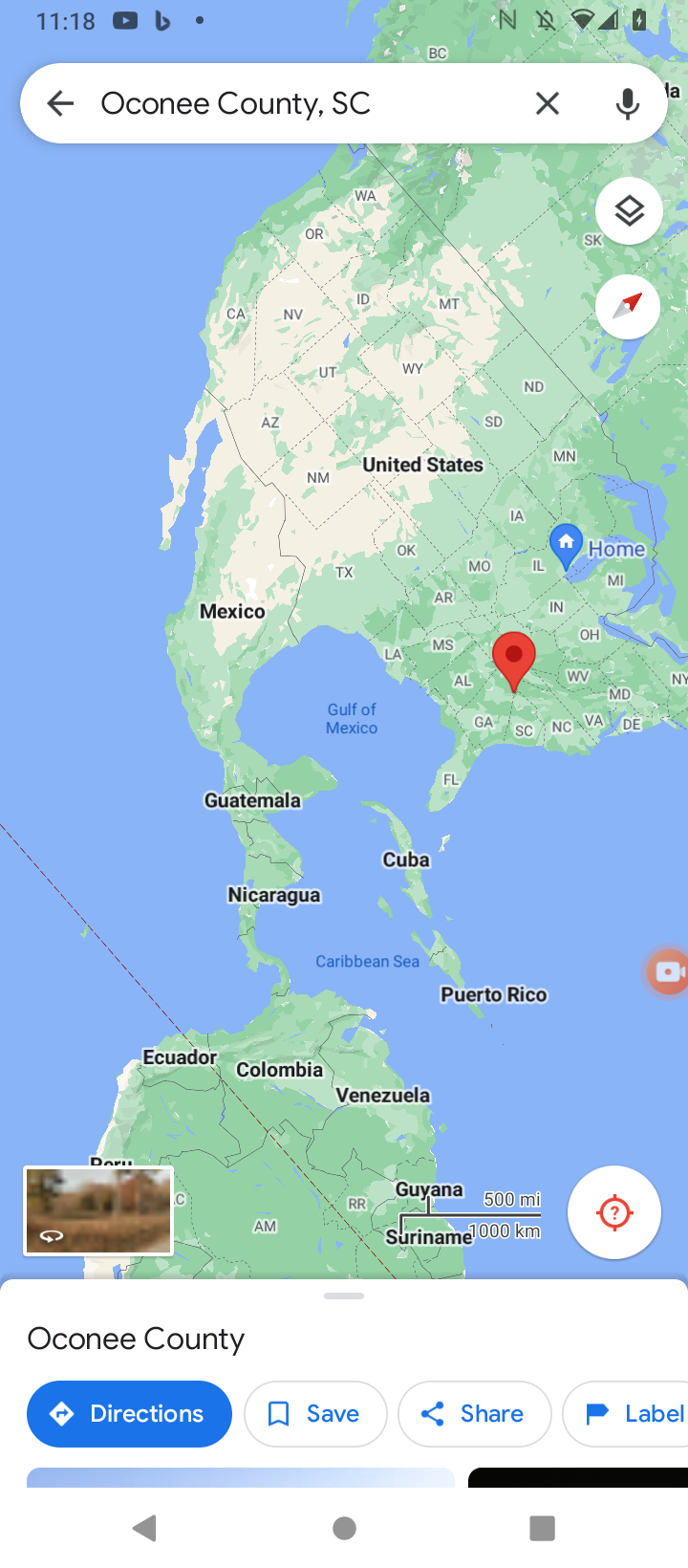This detailed image is a screenshot of Google Maps on a mobile phone, showing a search for Oconee County, South Carolina. The large, central portion of the screenshot displays a map of the United States, including parts of Canada, Mexico, Central America, and northern South America. The map is tilted, revealing labeled countries such as Ecuador, Colombia, Venezuela, Guyana, and Suriname, alongside notable bodies of water like the Gulf of Mexico and the Caribbean Sea. Each U.S. state is labeled with its two-letter abbreviation, with some exceptions. A red pin marks Oconee County in the Southeastern U.S., between Georgia and South Carolina, while another pin shows the user's home location near the Great Lakes, close to Illinois. The time shown on the phone is 11:18, with visible notifications from YouTube and another app, a strong Wi-Fi signal, and a charging battery. The search bar at the top clearly reads "Oconee County, South Carolina," and at the bottom of the screen, there are options to get directions, save, share, or label the location.